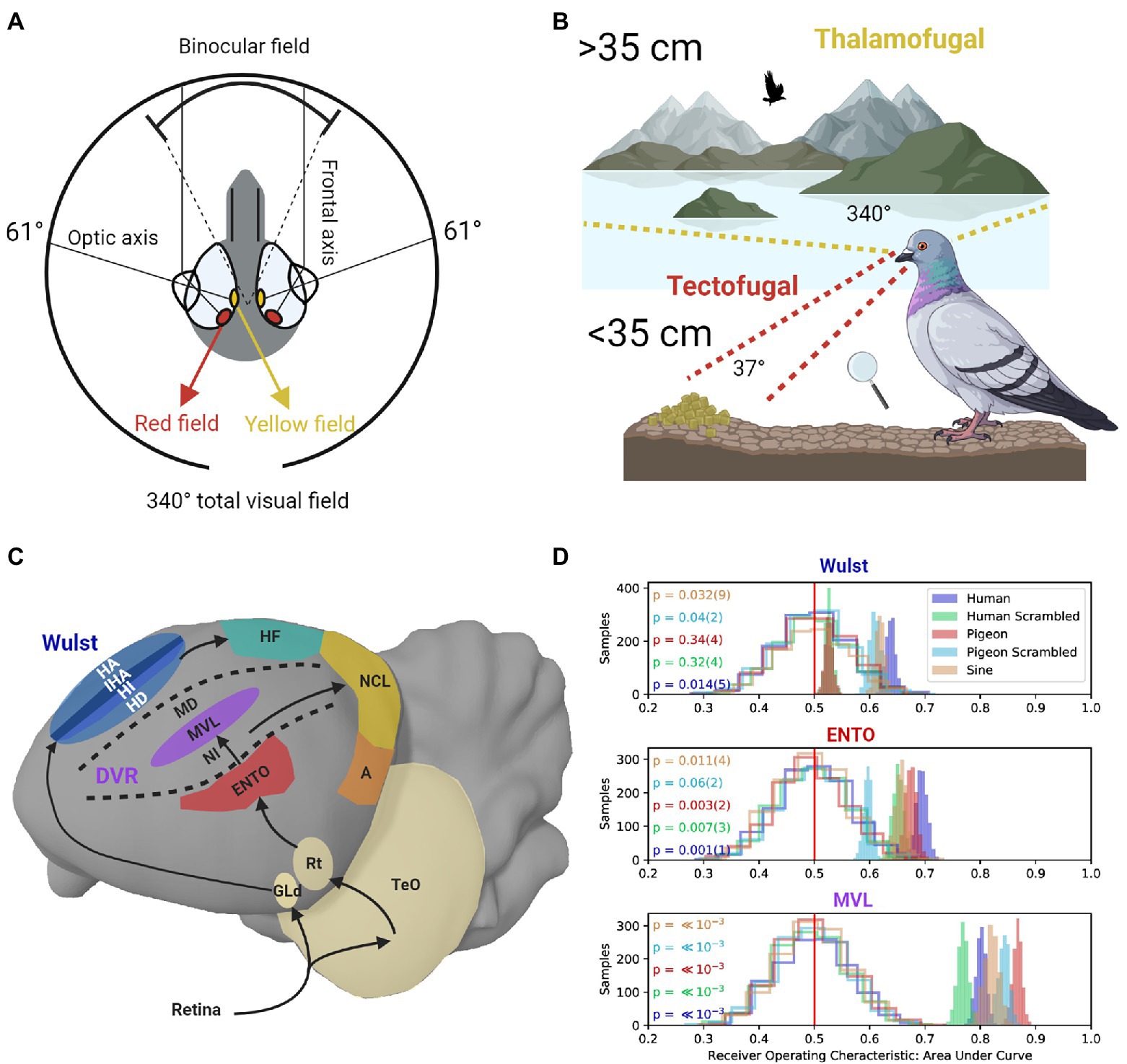The detailed image depicts a series of scientific diagrams and graphs illustrating the visual fields, brain structures, and neural pathways of birds, focusing specifically on pigeons. 

In the top left, there is a labeled diagram showing a circle with annotations: "Binocular Field" above it and "340 Degrees Total Visual Field" below, detailing the extensive visual range of birds. Inside the circle, terms such as "Optic Axis" and "Frontal Axis" are noted along with colored arrows indicating directional fields: a red arrow pointing down-left marks the "Red Field," and a yellow arrow pointing down-right marks the "Yellow Field." Central to this diagram is a gray sphere with a smaller sphere connected at the top.

The top right section features an illustration of a pigeon looking downward, with a scenic background including an eagle, mountains, and a lake. Here, visual markers extend from the pigeon’s eyes, labeled to show specific viewing angles and distances: "Tectofugal" and "Thalamofugal," with measurements indicating less than 35 centimeters or 37 degrees. 
 
In the bottom right corner, three graphs plot data with a legend identifying different lines: the purple line represents "Human," the teal "Human Scrambled," the red "Pigeon," the blue "Pigeon Scrambled," and the beige "Sign." These graphs are titled "WOLST," "ENTO," and "MVL," and collectively captioned "Receiver Operating Characteristic Area Under Curve," showing distinct patterns across the different subjects studied.

Adjacent to these graphs, a diagram of a bird's brain (or eye structure) is marked with multiple colored regions. "WOLST" is the header. Various regions are identified: a blue area labeled "H-A-I-H-A-H-I-H-D," a central purple region titled "MVL," a red lower area called "ENTO," another blue area to the right named "HF," a yellow region marked "NCL," and an orange section labeled "A." This structure connects to a larger gray mass that links to a beige mass labeled "TEO."

This comprehensive visual map and dataset articulates how pigeons perceive their environment, detailing both their visual fields and the specific brain regions involved in processing this sensory information.